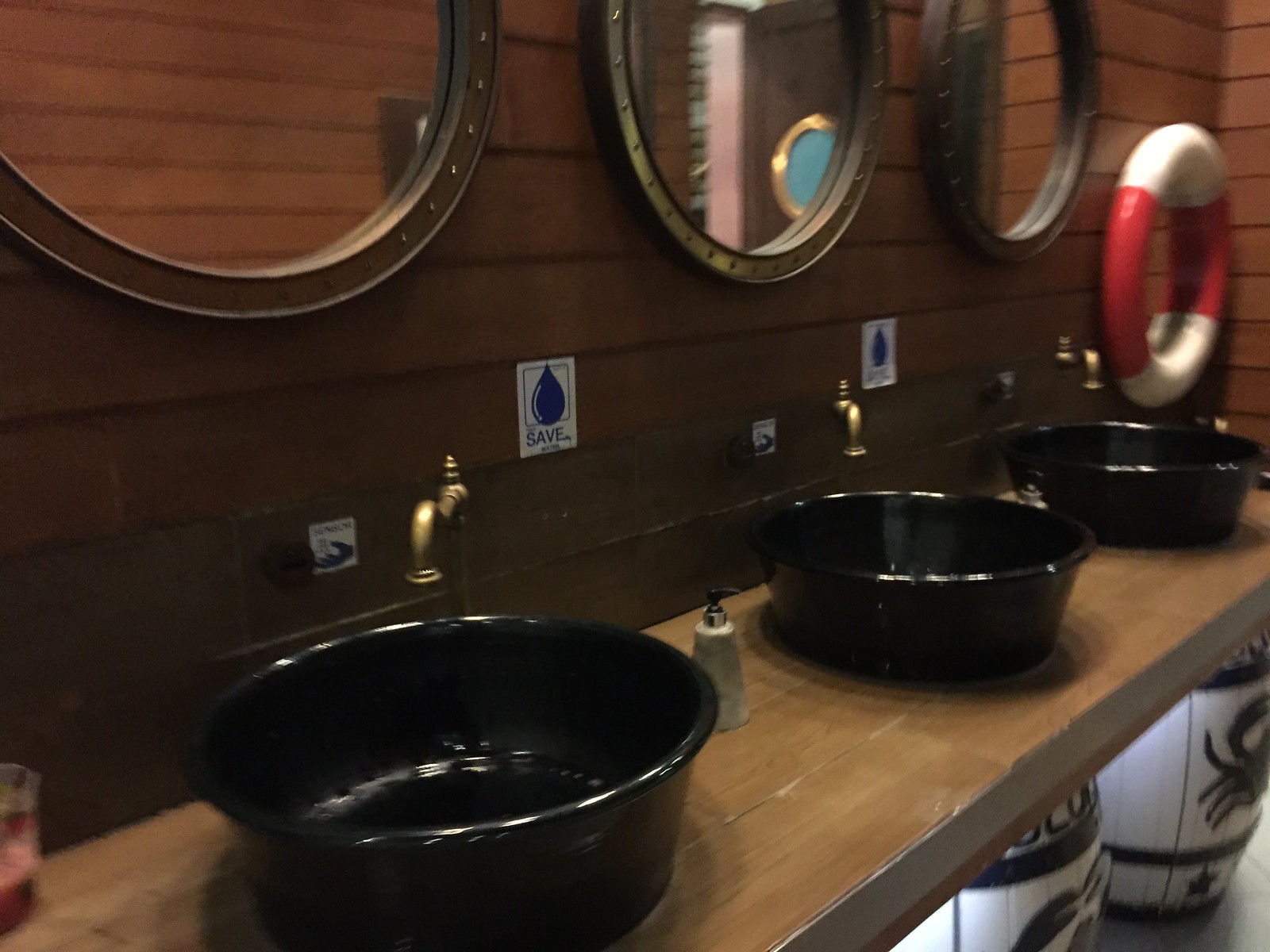This image is of a nautical-themed bathroom featuring a variety of intricate design elements. The walls are a dark brown paneling, reminiscent of ship interiors, providing a rustic, oceanic atmosphere. Central to the image are three black bowl-shaped sinks, each poised elegantly upon tan wooden countertops. Supporting these countertops are white and blue barrels adorned with blue crab designs, acting as unique sink legs. Each sink is furnished with a bronze-gold faucet, exuding an elegant touch. Above the sinks are three circular mirrors with tan borders dotted with small accents, resembling portholes on a ship. Between each sink, there are white signs with blue water droplets and the word "SAVE," alongside hand washing stickers, reinforcing the cleanliness theme. Soap dispensers are conveniently placed on the counter. To the right, a red and white life ring adds to the maritime décor, tying the theme together seamlessly.